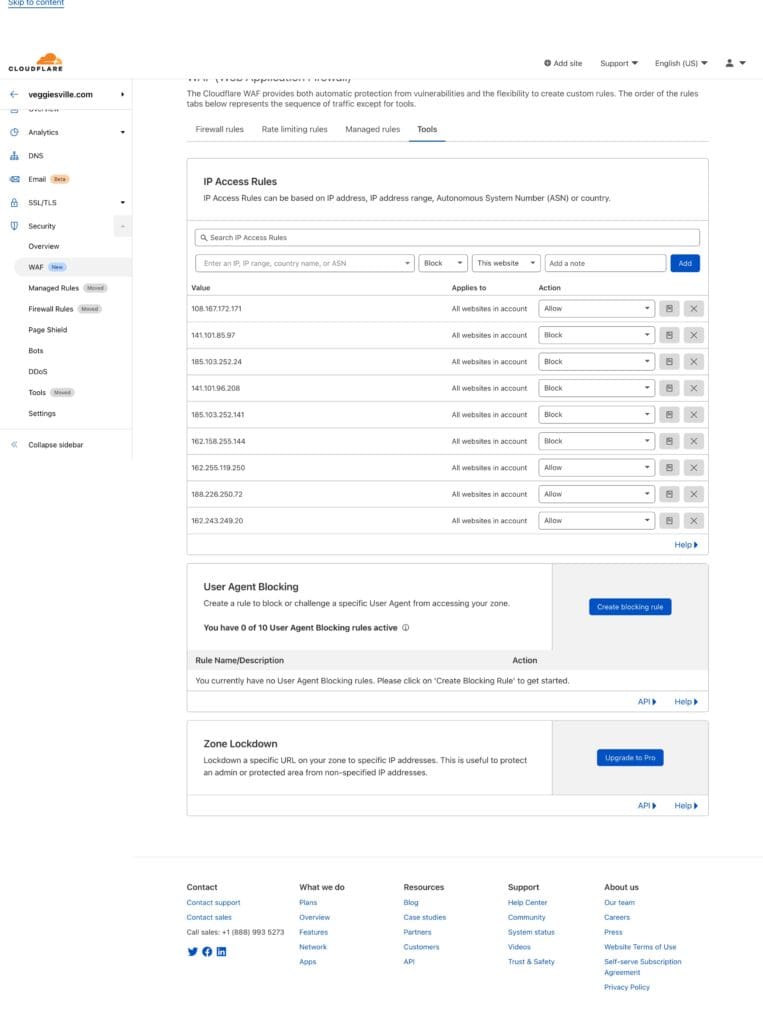The screenshot depicts a user interface, likely from a web-based application or dashboard. On the right-hand side, there is a section that includes an option to "Add Title" or "Add Like," both in English, followed by "(US)" to denote the language and region. Next to these options is a profile symbol, suggesting user account settings or profile management.

Below this, the screen shows a heading for "IP Access Rules," followed by a table. The table includes columns with headers such as "Value" and "Action." In the "Action" column, there are icons: a checkbox and a square with an 'X,' likely representing different actions that can be taken on the listed IP rules. 

Further down, there are sections titled "User Agent Blocking" and "Zone Lockdown," indicating more advanced security configurations.

At the very bottom, there are navigational links grouped under headings like "Content," "What We Do," "Resources," "Support," and "About Us." Each of these headings has a list of sub-links beneath them. All links are styled in blue, indicating they are hyperlinks, except for one link under the "Content" section, which is in a different color, possibly signifying it is either currently active or unavailable.

This detailed layout provides a comprehensive view of the various settings and navigation options available to the user.